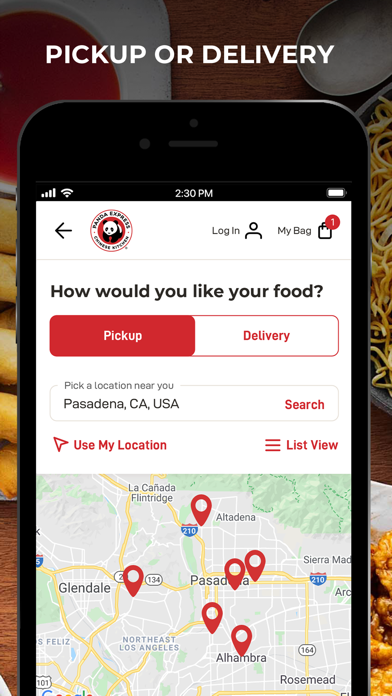This is a detailed caption for an image depicting a screenshot of an advertisement for Panda Express, focusing on their pickup or delivery options:

The image is a screenshot of an advertisement from Panda Express, showcasing their options for pickup or delivery services on a smartphone interface. The bottom half of the image consists of a black smartphone, with the screen displaying the advertisement. At the top of the smartphone screen, the time is shown as 2:30 p.m., and the battery icon in the top right corner indicates a full charge.

The main section of the screenshot prominently features the Panda Express logo located in the top left corner. The logo consists of a black and white panda inside a red circle, with the words "Panda Express" circling around it. Next to the logo, there's a login button and a shopping bag icon with a red circle containing the number one, indicating there is one item in the user's bag.

The advertisement poses the question, "How would you like your food?" providing the options for "Pickup" or "Delivery". Directly underneath, it instructs users to "Pick a location near you," with an example location of "Pasadena, California, USA" listed. There is a search button available for users to find nearby Panda Express restaurants, along with an option to use the device's location for convenience.

Additionally, the interface offers a list view option on the right-hand side and displays a map at the bottom, marked with various Panda Express locations in the specified area.

This cleaned-up, detailed caption effectively describes the image content and the functionalities presented within the app interface.